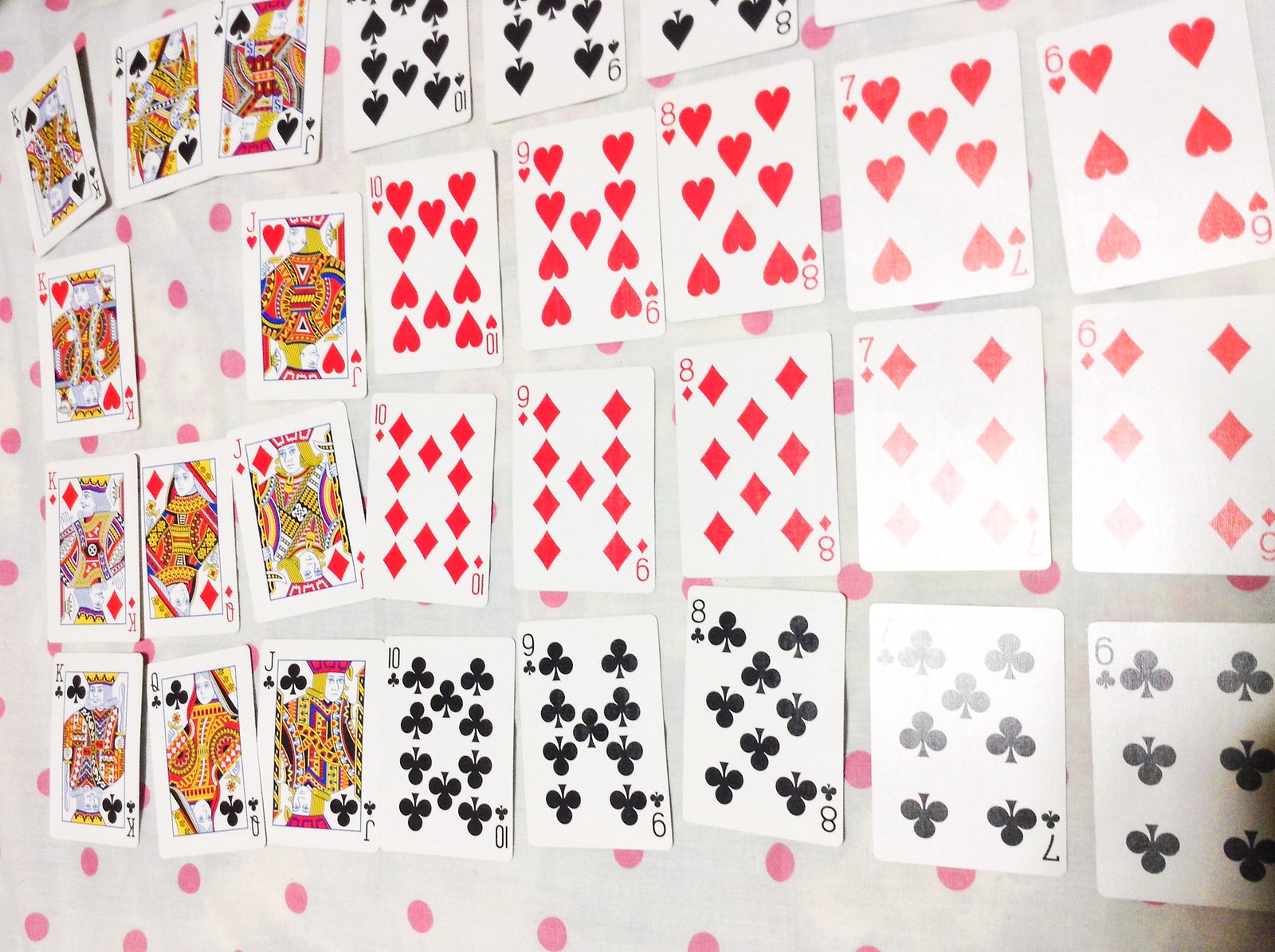The image showcases an array of playing cards meticulously arranged on a table, each card clearly rectangular and thin. The cards are organized into four sequential rows, extending beyond the visible frame. 

In the first row, the cards are ordered from the King of Spades down to the Eight of Spades, with the corner of the next card barely visible. The second row begins with the King of Hearts and follows through the suit in descending order. Similarly, the third row starts with the King of Diamonds and continues, with the last visible card being the Six of Diamonds. The fourth row starts with the King of Clubs and proceeds, ending visibly at the Six of Clubs. 

The table surface under the cards is covered with a white fabric adorned with pink polka dots, adding a whimsical background. There is a noticeable glare from what appears to be a camera's flash, affecting the area around the Seven and Six of Diamonds, as well as the Seven and Six of Clubs.